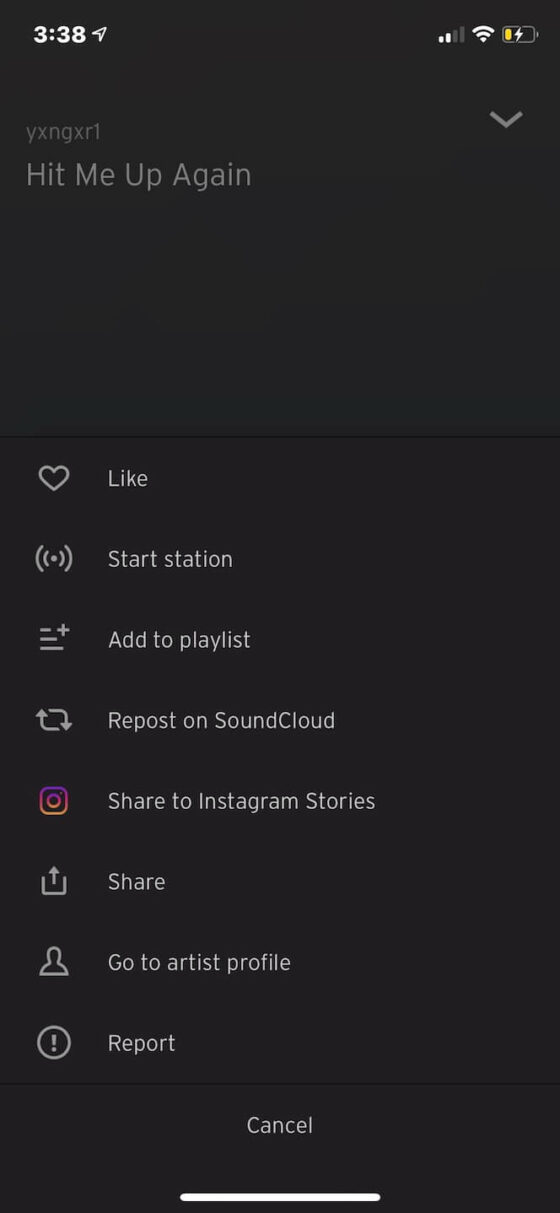A closely cropped screenshot from a smartphone depicts a social media account on a music-sharing platform, possibly SoundCloud. The device's status bar indicates it is 3:38, showing a few signal bars, connected Wi-Fi, and low battery with Power Saving Mode enabled. The account user, identified by the username "yxngxr1," appears to have a tagline or status message saying, "hit me up again." A dropdown arrow is situated next to the username, indicating more options might be available.

Beneath the username section, various interactive options are listed: "Start Station," "Add to Playlist," "Repost on SoundCloud," "Share to Instagram Stories," "Share," "Go to Artist Profile," and "Report." Notably, the Instagram icon is highlighted in color, though it is unclear if it is being actively selected. At the bottom of the interface, a "Cancel" option is present, suggesting the user is in the midst of deciding their next action. The context implies "hit me up again" could either be a personal tagline of the user or the title of a song they are engaging with.